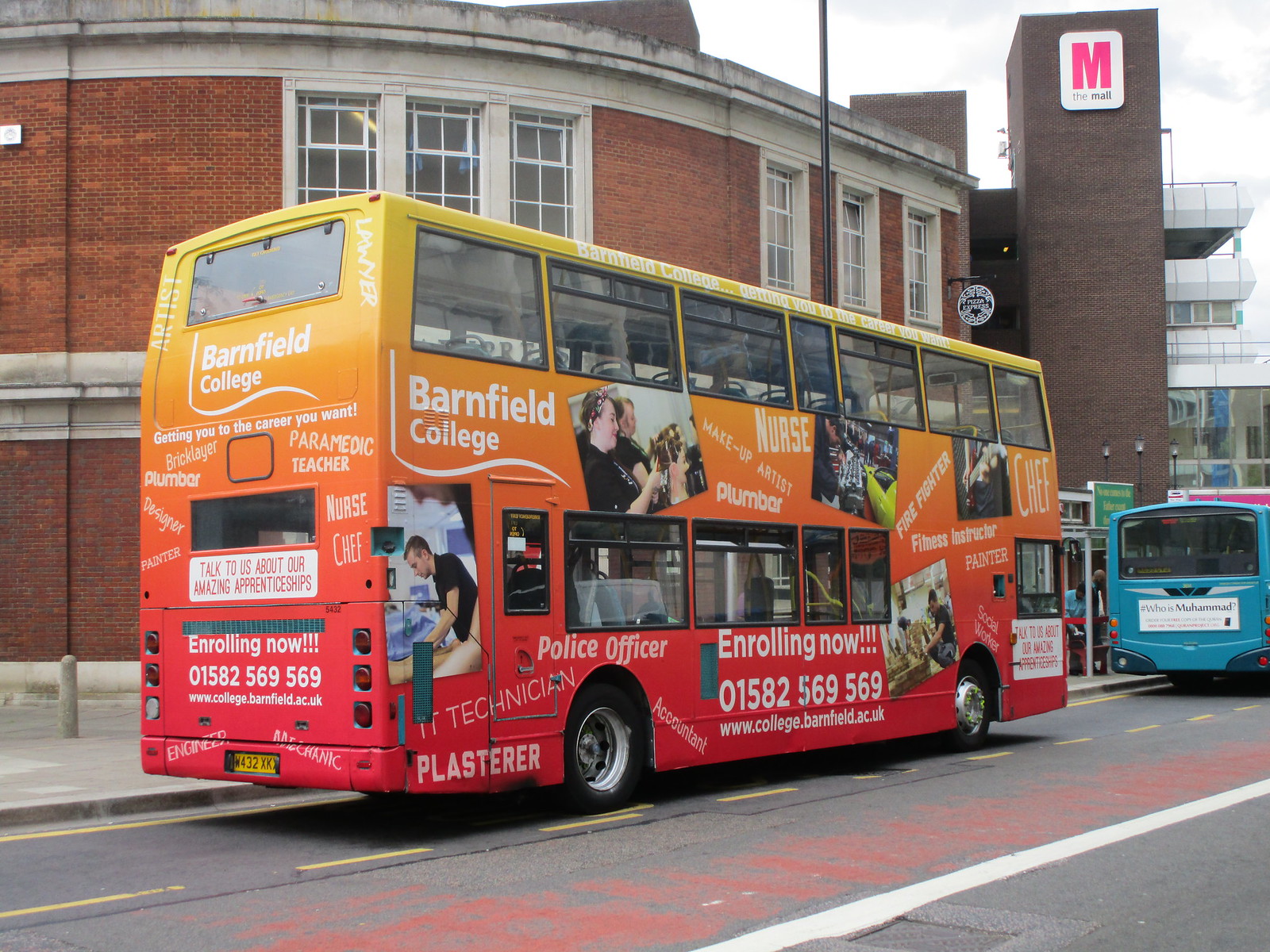The image features a vibrant, double-decker bus prominently situated on the left-hand side of a road marked with both a white solid line in the middle and a dark yellow line on the left side. The bus itself displays a striking ombre color scheme, transitioning from yellow at the top to orange and then to red at the bottom. This multicolored bus is adorned with numerous advertisements for Barnfield College, promoting various careers such as nurse, paramedic, teacher, chef, and police officer, among others. The side of the bus also features large text stating "Enrolling Now!" and includes the phone number 01582 569 569.

In the background, a tall brown tower with a logo "M" on the top is visible to the right, while a brown building with white windows lines the sidewalk. Additionally, a blue-tinged vehicle, possibly another bus, is positioned in front of the double-decker. In the distance, a few people are sitting at a bus stop amidst more buildings. The detailed urban setting is complemented by a clear view of the street in the bottom right corner of the image.